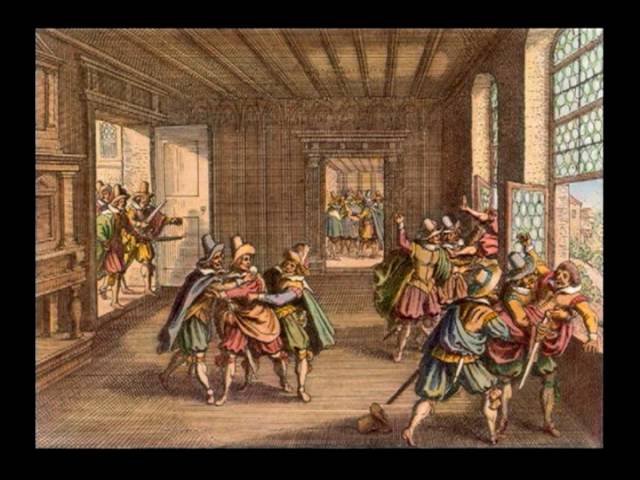The artwork depicts a bustling scene in a large, welcoming hall, characterized by its open window and light brown wooden interior. The room is filled with dynamic conflict, showcasing a detailed historical scuffle involving around 12 to 13 individuals. The men, adorned in colorful robes resembling those of court jesters, and tall wide-rimmed hats, are seen in various confrontations. 

In the center, three main groups of men engage in heated exchanges. A central figure is being restrained by two others, while on the right side, another group wrestles as one man’s hat lies on the ground and another wields a sword. Adding to the chaos, two individuals are depicted trying to throw a struggling man out of the window. 

Further left, through an ajar door, two more men armed with swords are entering the scene. In the background, an additional open door reveals a crowd engaged in discussion. The artwork, possibly from the 17th or 18th century, conveys a sense of urgency and turmoil within its grainy yet vividly colored depiction, framed by a striking black border.